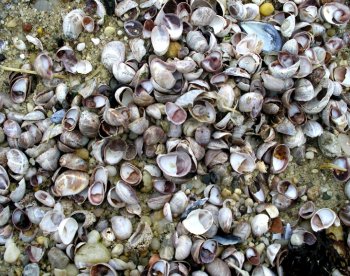The image showcases a densely packed collection of seashells, predominantly the outer shells of mussels, strewn across what appears to be a sandy shoreline. The shells are of various colors including white, blue, and a few orange-yellow ones, creating a visually striking mosaic against the soft, possibly wet, sand. Some small pebbles are interspersed among the shells. The shells, numbering around fifty, are both open and closed, and appear jumbled and heaped on top of each other, covering nearly the entire frame. There is a discernible spot in the upper left corner where the sand is visible through the sparse shells, and a similar sandy gap and a black mass—possibly a foot or kelp—at the bottom right corner, further emphasizing the natural beach setting.